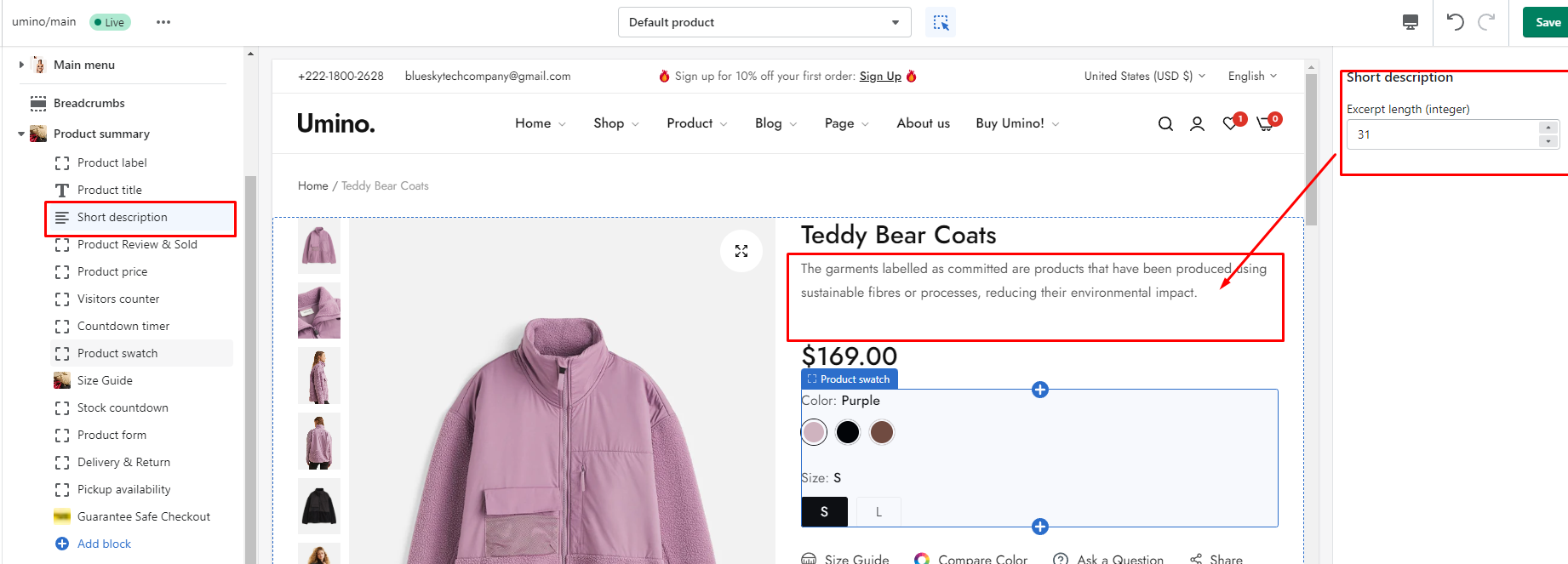This image is a screenshot of a web page from the website Yumino, showcasing a teddy bear coat for sale. The page layout features a vertical main menu in the left column, which includes the following sections: breadcrumbs, product summary, product label, product title, a highlighted short description, product review, items sold, product price, visitor counter, countdown timer, product search (also highlighted in gray), size guide, stock status, countdown, product form, delivery and returns information, pickup availability, guarantee of safe checkout, and an advertisement block.

At the forefront is an image of the featured teddy bear coat, which is pink. The page also includes five additional photographs of the coat. The garment label emphasizes the company's commitment to sustainable fibers and processes, aiming to reduce the environmental impact of their products.

The short description box features an excerpt with a length of 31 characters. The pink teddy bear coat is priced at $169.